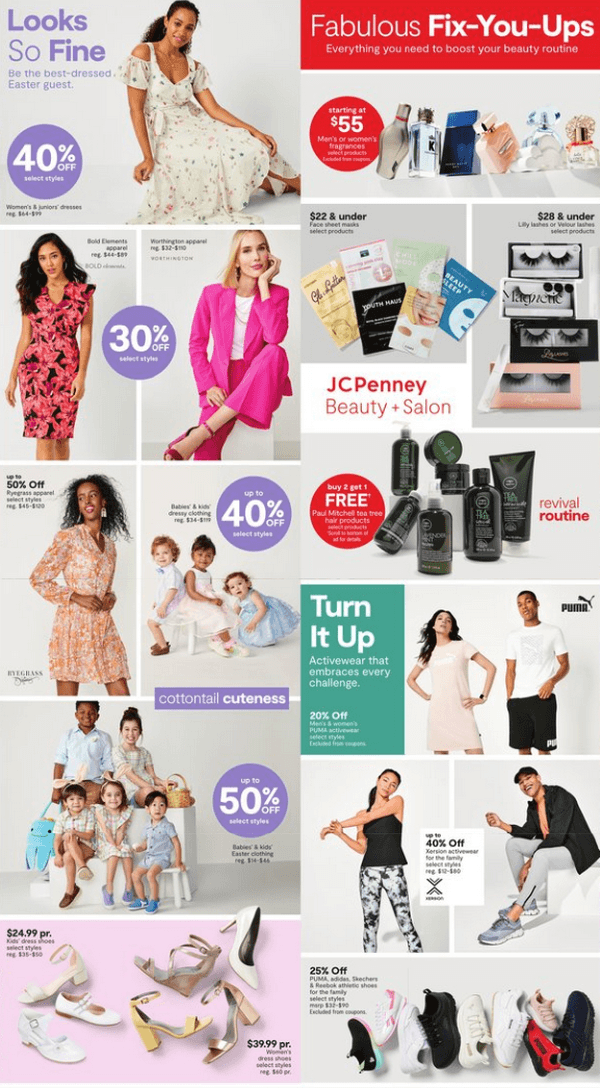This is a JCPenney sales flyer that captures attention with its full-color presentation. Designed to be either a printed flyer available in store or a piece of promotional mail, it features vibrant accent colors: violet, cherry red, and teal. At its center, a dedicated box prominently announces “JCPenney Beauty Plus Salon,” clearly identifying the retailer. The flyer is compartmentalized into 16 distinct boxes, each showcasing various products with brief descriptions. The assortment includes images of dresses, business attire, false eyelashes, skincare products, athletic wear, dressy shoes, and athletic footwear. Each section reflects different store departments, offering a comprehensive snapshot of available merchandise. Discount percentages range from 30% to 50% off, though not all boxes display a discount figure.